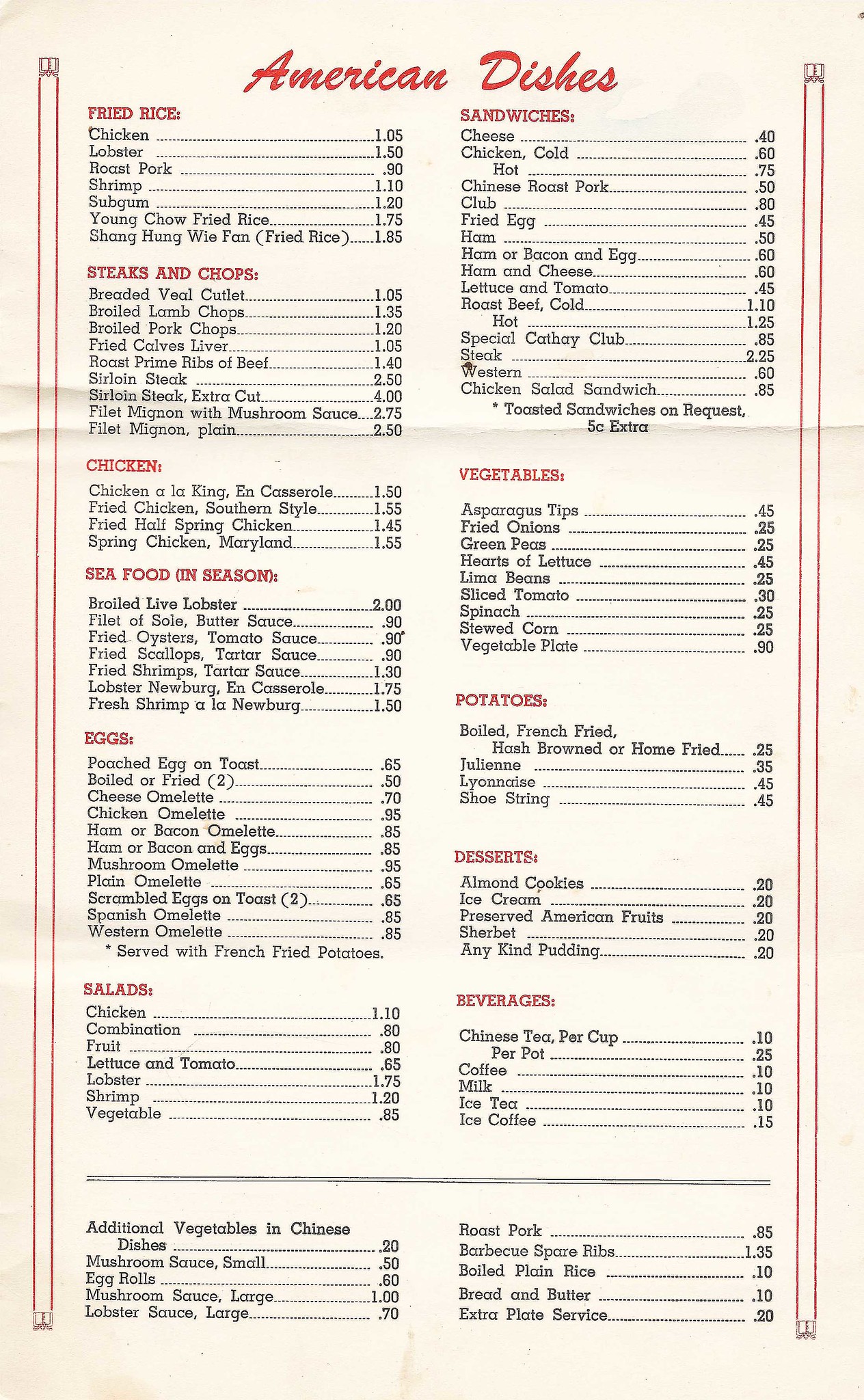The image showcases a vintage menu titled "American Dishes," printed on an off-white, slightly yellow piece of paper that bears the marks of a previous tri-fold, though it now lies flat. The menu's title, "American Dishes," is elegantly presented in a cursive red font at the top. Further down, the menu is structured with headings, each in uppercase red text, denoting various categories of dishes. These categories include "Fried Rice," "Steaks and Chops," "Chicken," "Seafood in Season," "Eggs," "Salads," "Sandwiches," "Vegetables," "Potatoes," "Desserts," and "Beverages," followed by additional extra dishes listed at the bottom.

The design features two parallel red lines running down each side, forming a border that frames the contents symmetrically. Each dish under the respective headings is listed in black text, accompanied by a series of dots that lead the eye to the price, positioned on the right-hand side of each listing. The menu does not specify the currency for the prices. Additionally, the content is organized into two main columns, enhancing readability and structure. The overall aesthetic exudes a sense of classic American dining, with an emphasis on clarity and tradition.